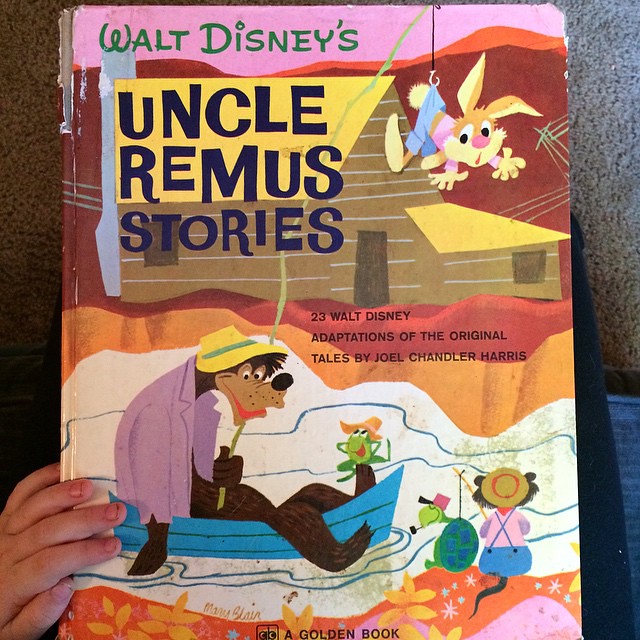The image depicts a well-worn, full-colored hardcover book titled "Uncle Remus Stories," featuring 23 Walt Disney adaptations of the original tales by Joel Chandler Harris. The cover, which shows significant wear with a partially torn spine and rip on the upper right-hand edge, sits against a mottled brown and white background, likely a wall. Held up by a woman’s right hand with long fingernails, the book is prominently featured. 

The title “Walt Disney's Uncle Remus Stories” is printed at the top in green and large dark blue letters left-aligned. Central on the cover is a vivid illustration with multiple Disney characters in various vibrant colors. Dominating the scene are a bear clad in a purple shirt and yellow hat, along with a frog in a straw hat, both sitting in a blue canoe on a white river. To the side, a bunny, appearing to be Briar Rabbit, dangles from a string attached to his pants in the upper right corner of the cover. Adding to the detail, other characters such as a turtle and a muskrat are seen fishing, surrounded by elements in reds, pinks, oranges, and yellows. At the bottom, the book is identified as "A Golden Book."